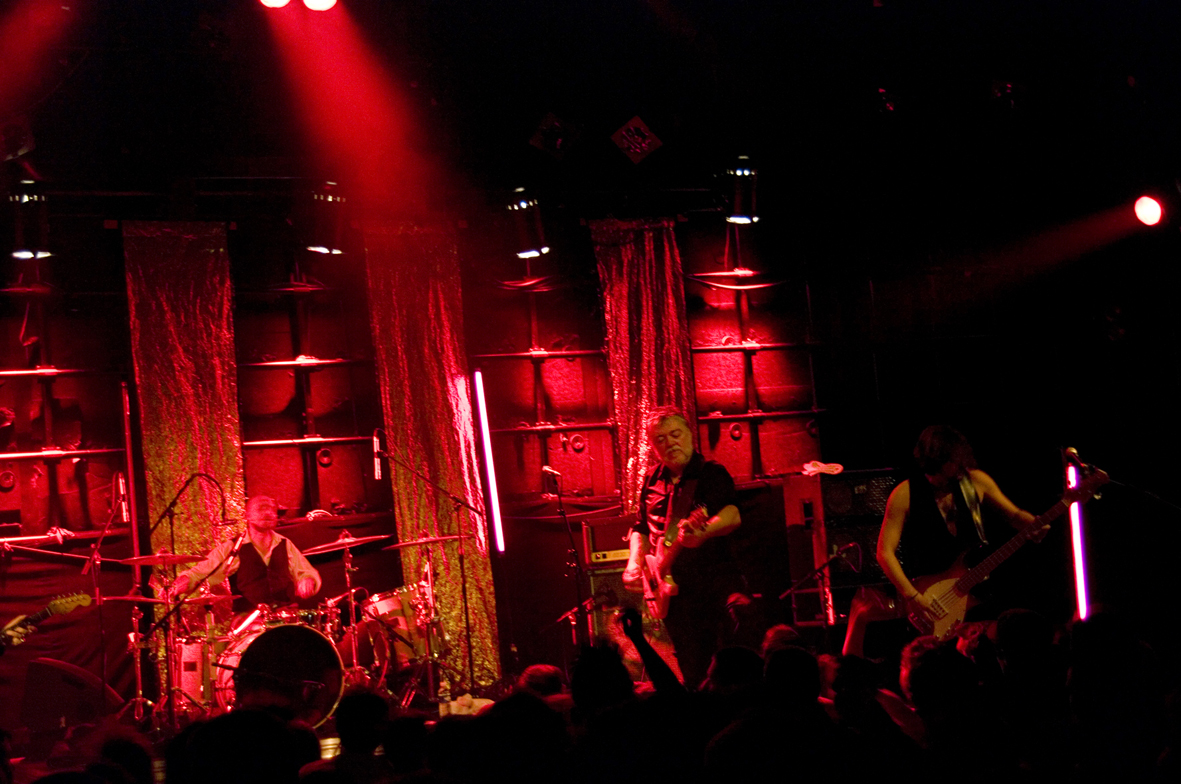This interior photograph captures a dynamic moment during a rock band's performance on stage at a nightclub or music venue. The band, bathed in intense, filtered red strobe lighting from above, includes a drummer positioned on the left, energetically playing his drum set, and two guitarists. The central guitarist, an older man with gray hair and a beard, dressed in a black t-shirt and pants, is angled three-quarters to the left, strumming his guitar with focused intensity. To his right, another guitarist, leaning slightly forward, is also engrossed in playing, though his face and head are obscured in the dark lighting. He wears a dark sleeveless shirt and, like his bandmate, grips the guitar's neck with his left hand while playing with his right. The stage is situated in a high-ceilinged room accentuated by additional red lighting against the back wall, which is adorned with long, decorative panels in gold hues that create an ambient backdrop. Visible in the upper right area of the photograph is a white strobe light aimed at the band. In the foreground, the silhouettes of audience members reveal their attentive engagement with the performance, their darkened figures contrasted against the vivid illumination enveloping the musicians.